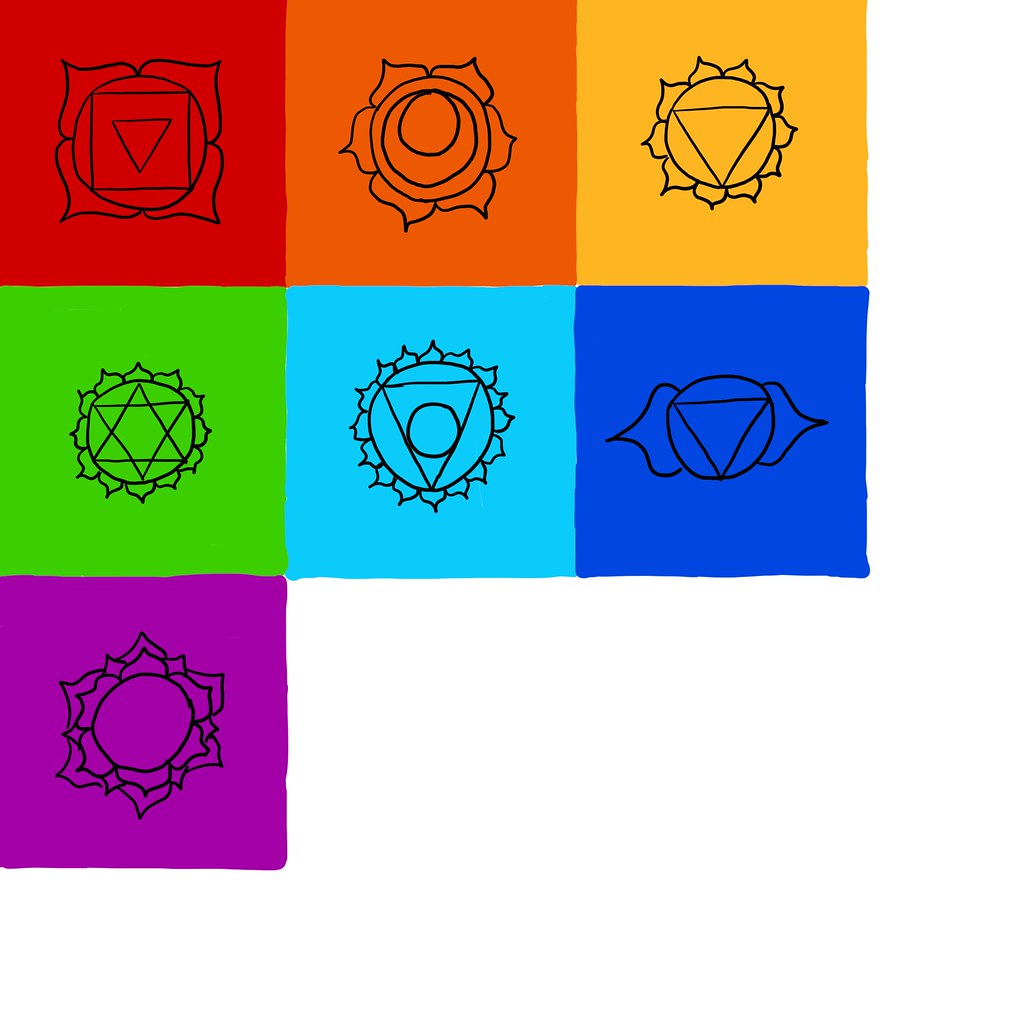This is a multi-color print piece comprising a 3x3 grid of equal-sized squares, though the bottom row is incomplete, featuring only a square on the far left and right. Each square is uniquely colored and adorned with geometric floral designs, predominantly incorporating triangles. Starting from the top left and moving right, the colors are red, orange, yellow, green, blue, light blue, dark blue, and purple. The red square in the top left displays a rose-like figure, advancing to an orange square with a rounded flower. The yellow and green squares both have sunflower-like designs. The turquoise square features intricate layering with a circle within a triangle within a sunflower. The royal blue square presents a triangle inside a circle with wing-like extensions. Lastly, the purple square contains another sunflower-like motif. The image provides an overarching rainbow of colors enriched with detailed geometric floral patterns.